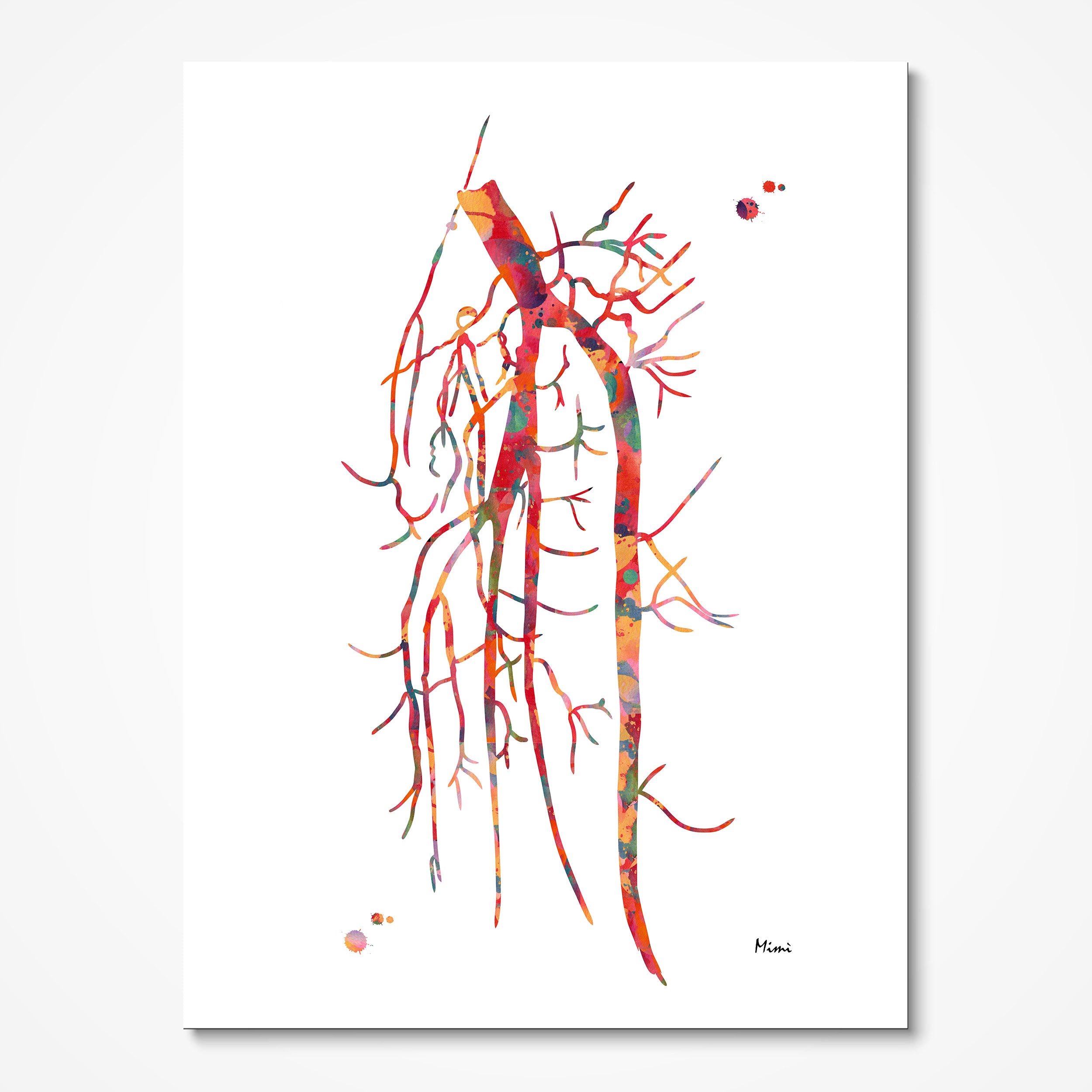This detailed description captures the essence of the painting using the most repeated and emphasized elements from all three captions:

The image is of a painting displayed on a white wall, showcasing a vertical rectangle orientation. The painting features an intricate and colorful root system, reminiscent of tree roots or veins, expressed in a stylized, almost abstract manner. At the center is a large root system, from which several smaller root systems extend outward, thinning as they move away from the main body. One root system on the left appears to ascend higher than the central one. The roots blend in a hodgepodge of vivid hues, including red, green, yellow, pink, and blue, creating a watercolor-like effect, as if the colors were dripped and allowed to mix naturally. Scattered around the bottom left and upper right corners are clusters of small, colored dots. The artist's signature, reading "Mimi," is found at the bottom of the painting in black ink, adding a personal touch to this vibrant and dynamic piece.